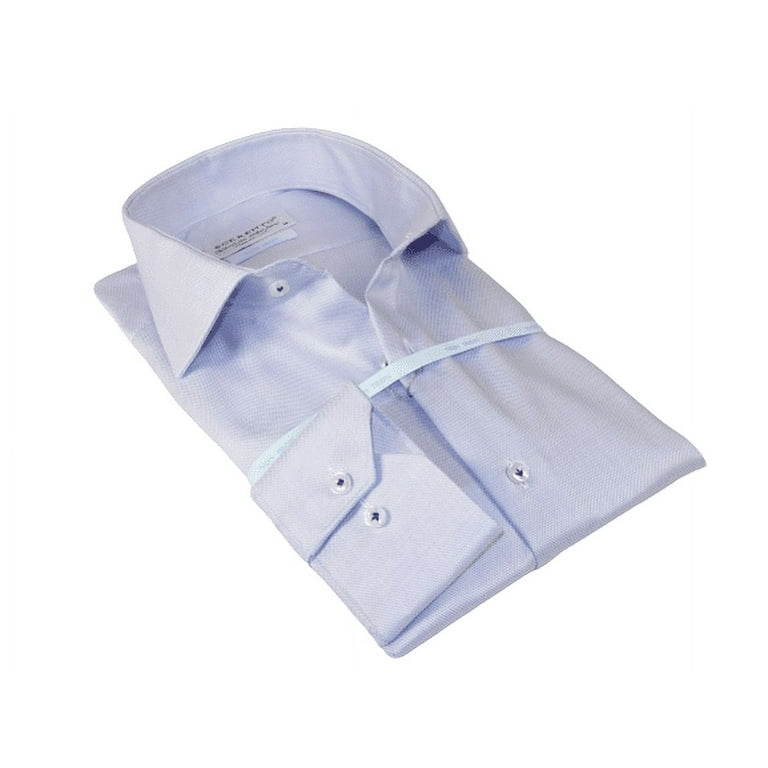This detailed photograph captures a neatly folded, light blue men’s dress shirt, commonly seen in retail settings or after laundry services. The shirt is arranged into a precise rectangular shape, with the collar standing stiffly upright and the fold lines meticulously evident. A light blue ribbon encircles the shirt, suggesting it’s new or prepared for sale; the ribbon has writing that is too blurred to read. The fabric of the shirt appears to be either light cotton or a blend, characterized by fine horizontal lines.

Prominent features include a pocket on the left side featuring two small white buttons with dark blue thread, suggesting attention to design details. On the right side, there is a slight upward tilt to one of the visible buttons. The shirt’s overall structure is held together by the blue ribbon, with the collar facing upwards in the top left section of the image. The cuff of the left sleeve is folded over towards the center, showcasing two more buttons identical to those on the pocket.

The background of the photograph is plain, ensuring all focus remains on the shirt itself. Wrinkles cascade down both sides, more prominently on the right from the collar down to nearly the button’s edge, adding a touch of texture to the crisp presentation. Additionally, a tag is visible, although the specific details remain unreadable, indicating brand and size information likely intended for consumer knowledge. Overall, the image conveys a polished and professional impression of the dress shirt.